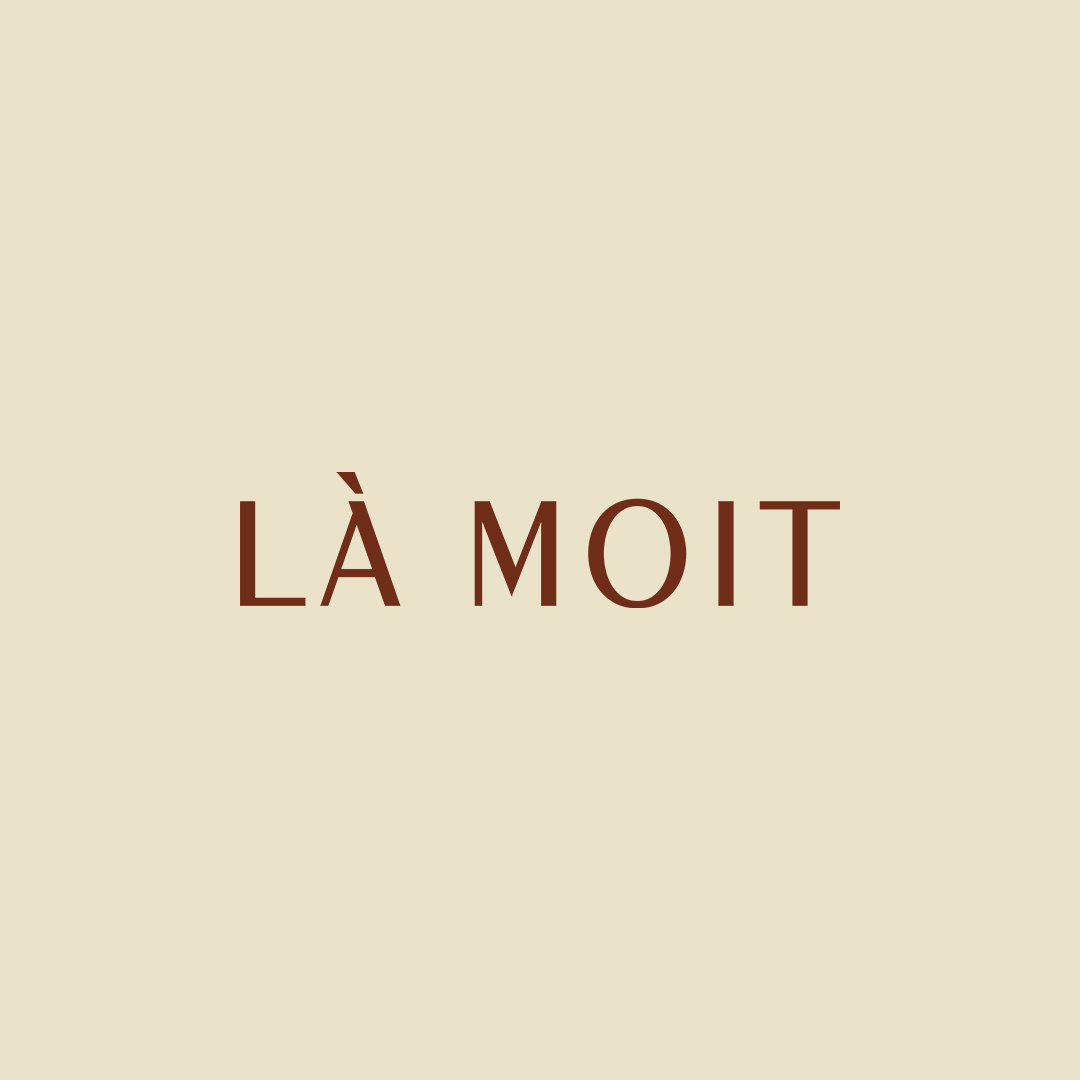The image presents a minimalist design featuring the potential branding for a company, label, or restaurant. Set against a solid beige background, the image is devoid of any objects, artwork or additional imagery, emphasizing simplicity and elegance. At the center of the background, the text "La Moit" is prominently displayed in a dark burgundy or brown-colored font. The characters include an international-style A with a grave accent, further suggesting a possible connection to another language or cultural aesthetic. The overall design is stark, with wide open spaces and no other elements, directing full attention to the central text, possibly indicative of high-end fashion or luxury branding.